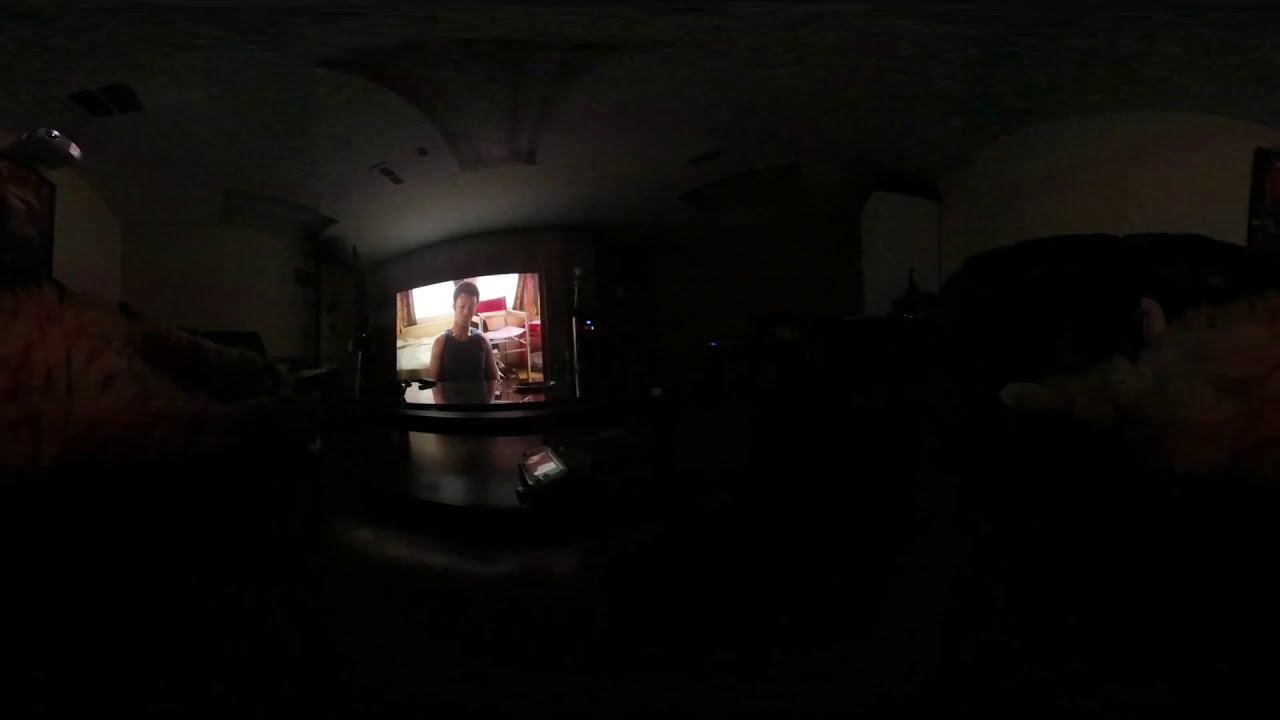This image captures a darkened indoor room, possibly taken at night, where the primary light source comes from an old big tube television slightly off-center to the right. The room’s details are mostly obscured by shadows, yet faint outlines of a couch, cushions, and a brown table can be discerned amidst the darkness. The TV screen displays a young African-American man, likely in his mid-20s, with short hair and a black tank top, looking slightly downward. He appears to be in a hospital room, as indicated by the hospital chair and bed, along with red curtains in the background. The TV screen also has a few green dots. A smartphone is visible on the table in the foreground. The illumination from the TV casts light onto a white ceiling with a distinct brown streak in the middle.